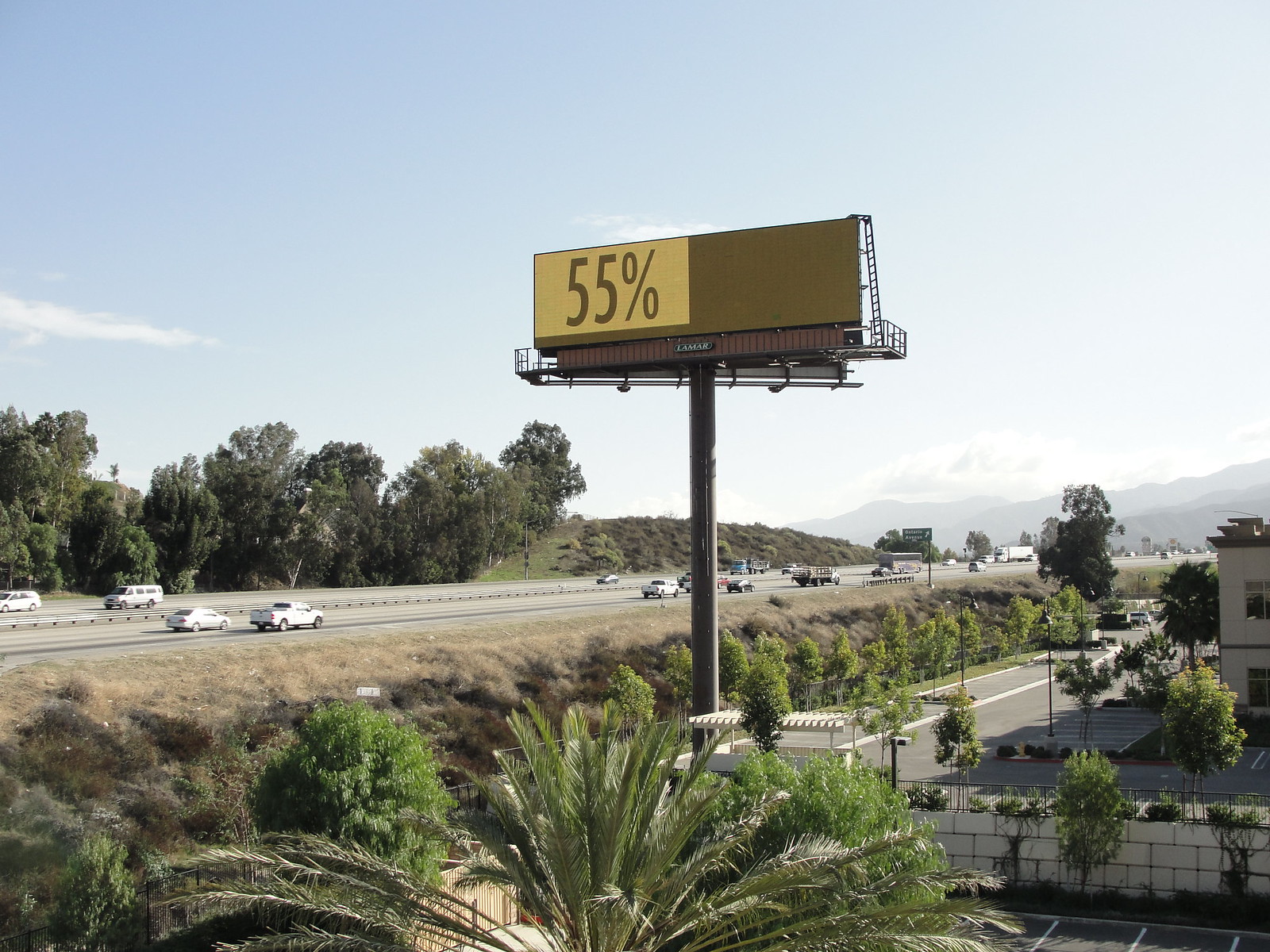The image depicts a billboard situated near a divided highway, prominently placed in the center of the frame. The billboard itself is structured on a pillar with a platform and ladder for maintenance. The left section of the billboard displays "55%" in dark brown lettering on a mustard yellow background, while the right section is solid dark brown. The scene is set during daytime with clear blue skies and a few clouds visible on the left. In the background to the right are snow-capped mountains, and a tree line runs along the left. The highway below, populated with various vehicles including cars, SUVs, and a cargo truck, wraps around the scene. In the foreground, a concrete block fence topped or flanked by bushes and the top of a palm tree can be observed, indicating an elevated viewpoint. The empty brown section of the billboard humorously signifies an incomplete message, metaphorically suggesting that only 55% of the advertising space is in use.